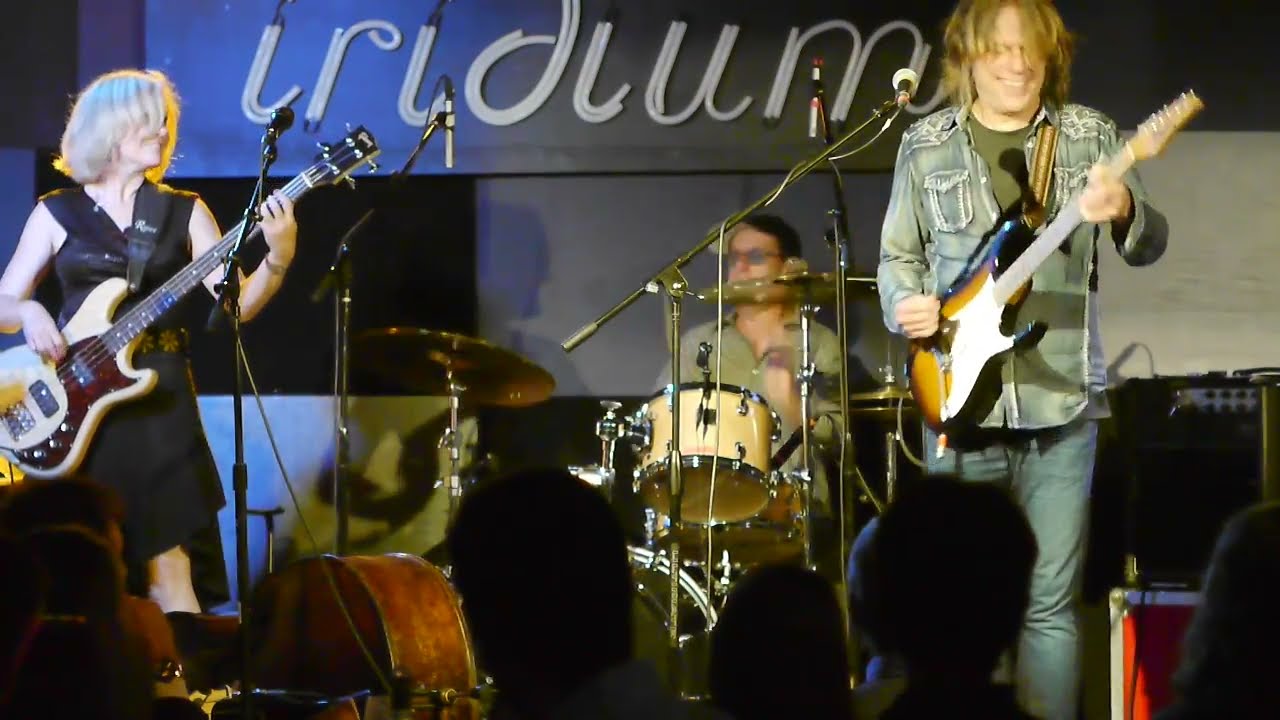The image captures a vibrant rock band performance at a venue with a cursive sign that reads "Iridium" in the background. The stage features three musicians: on the left, a blonde female guitarist plays a white electric guitar with brown accents, sporting bangs that partially cover her face and wearing a black dress. In the center, a male drummer in a light green button-down shirt and glasses energetically plays his drum set, partially obscured by microphone poles and a cymbal. On the right, the lead guitarist, a man with long, blondish hair, is caught in the moment of his performance—his hand on the multi-colored electric guitar is a blur of motion. He's dressed in a denim button-down shirt layered over a green t-shirt and jeans. The photo, taken from a few rows back, shows the musicians immersed in their music, suggesting the scene is a lively concert with an enthusiastic audience just out of frame.